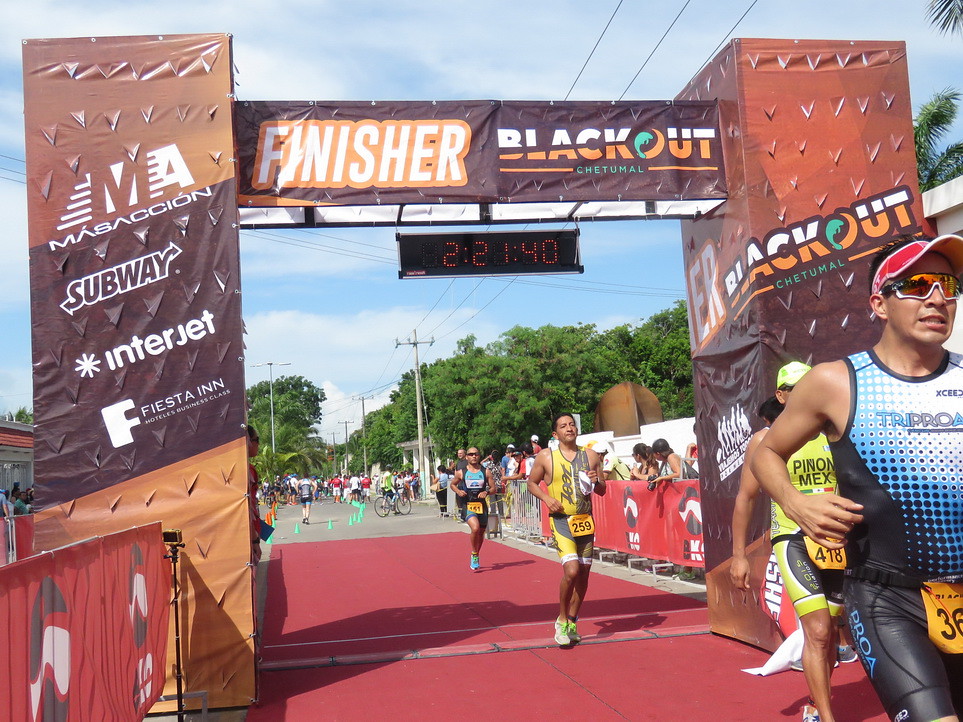The image captures the bustling scene at the finish line of a marathon event, marked by a prominent scaffolding archway draped with a brown tarpaulin adorned with sponsorship logos and event branding, specifically "Blackout Chetumal" in white and orange letters. At the top of the archway, a digital timer displays "2:21:40". Below, a red carpet accents the finishing area, flanked by two towers wrapped in fabric, each bearing additional sponsor logos such as Massa Sion, Subway, Interjet, and Fiesta Inn.

In the foreground, a determined runner in yellow and gray, wearing an orange bib numbered "259", has just crossed the finish line. Just behind him, another participant in yellow and black sporting the number "48" approaches the line. To the right, two more runners dressed in sports attire, one in black and blue with sunglasses and a vest, and another in yellow and black, stand observing the scene. Further back, more runners can be seen making their final strides towards completing the race.